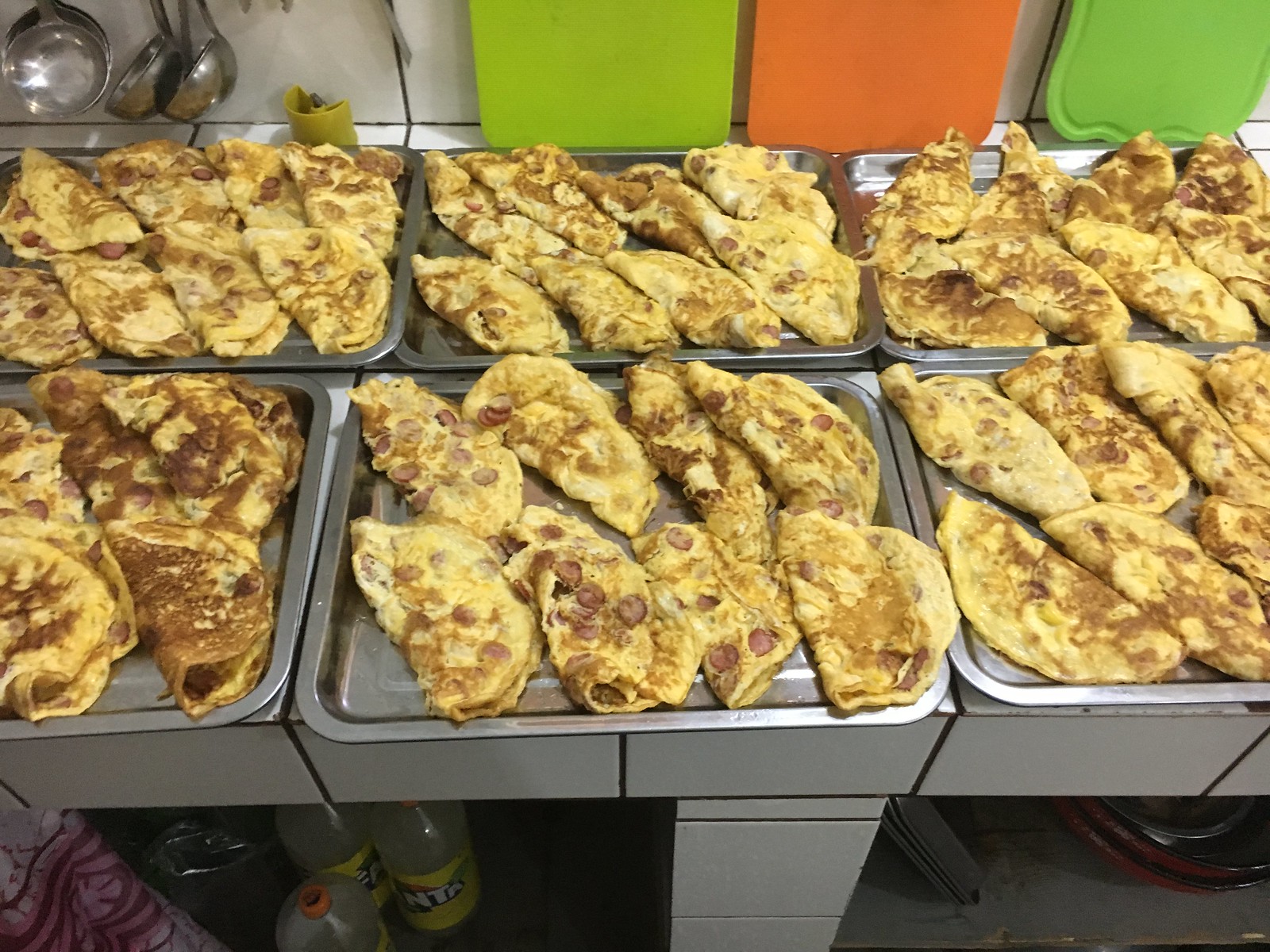This photograph captures a bustling kitchen setup, likely for a buffet line. The focal point is a series of six metallic trays, each meticulously arranged in two rows of three, covering the entire countertop. Each tray holds eight folded omelets, neatly arranged in semi-circular folds, with visible browned edges indicating some overcooking. The omelets exhibit a characteristic scrambled egg yellow color and are garnished with circular slices of meat, presumably sausage or hot dogs.

The counter surface is tiled in a clean white pattern, with open shelving below housing various kitchen essentials, including cleaning products and culinary tools. Visible items include two 2-liter bottles of Fanta Lemonade, a trash can, and an assortment of pots, pans, and bowls. A cloth can be seen on the bottom left.

In the background, large ladles and metal spoons hang from hooks against the wall, accompanied by three cutting boards in assorted colors—a lime green one, a vivid orange one, and a darker green, more rounded one—resting against the wall. The detailed setup showcases an organized kitchen meticulously prepared for a large-scale food service.